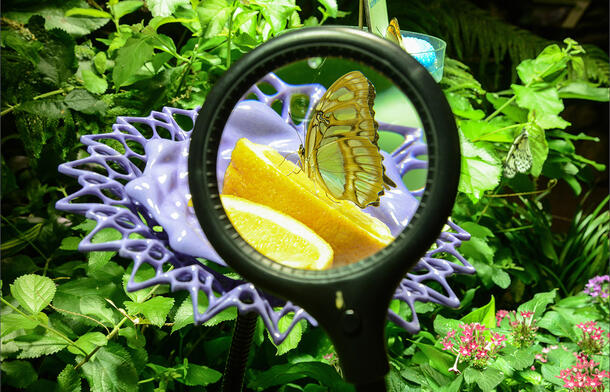In this detailed photograph set in nature, lush green foliage fills the background, interspersed with small pink and purple flowers in the lower right-hand corner. At the heart of the image, a black magnifying glass reveals a close-up of a delicate yellow butterfly with translucent wings edged in black, perched on a halved lemon. The butterfly appears almost iridescent under the lens, which clearly captures its intricate details, including its antennae. The lemon rests atop a peculiar, large purple structure that resembles a flower but has a shiny, webbed texture, suggesting it could be a butterfly feeder. Sunlight filters through, illuminating the scene and giving the entire composition a vibrant, lifelike quality. In the background, another faint image of a butterfly in a separate container adds a layer of depth and intrigue to this enchanting garden vignette.